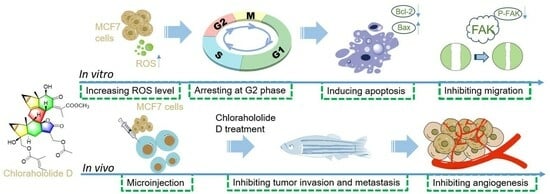This scientific illustration presents a detailed comparison of cellular processes in in vitro and in vivo environments, often found in educational materials. The top row, labeled 'in vitro,' begins with a depiction of MCF7 cells (resembling brown cookies) and follows a sequence with blue arrows indicating the corresponding stages. These stages include increasing Reactive Oxygen Species (ROS) levels, arresting at the G2 phase signified by a ring with segments labeled G1, S, G2, and M, inducing apoptosis, and inhibiting cell migration, marked by two disks with an arrow. The bottom row, labeled 'in vivo,' illustrates the biological effects of chlorohalolide D treatment via microinjection. This segment demonstrates the treatment's capacity to inhibit tumor invasion, metastasis, and angiogenesis, represented by images of blue blobs with brown dots, syringe, fish, and corresponding annotations.